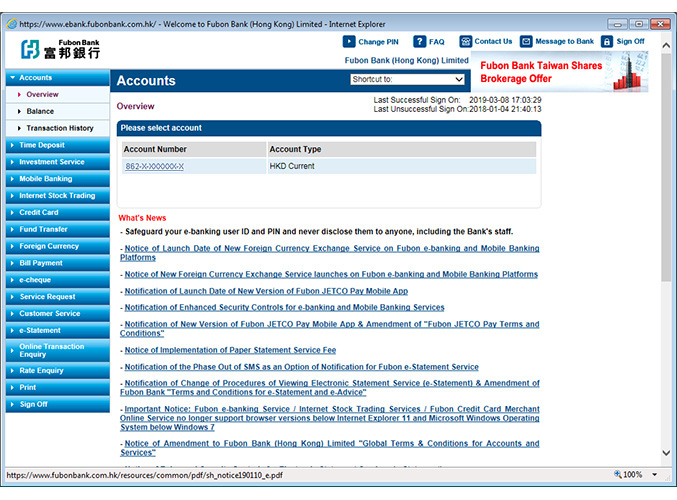The image shows a computer screen displaying the homepage of the Fubon Bank Hong Kong Limited website. The top of the screen features a gray bar that contains the website's name, followed by a welcome message that reads, "Welcome to Fubon Bank Hong Kong Limited." In the top right corner, there is a red square with an 'X' inside, which likely serves as a close button for the window or application.

Below the welcome message, "Fubon Bank" is prominently displayed along with a line of text, possibly written in Korean. A menu bar beneath this offers several options: "Change PIN," "Frequently Asked Questions," "Contact Us," "Message to Bank," and "Sign Off."

To the right, there is a vertical navigation column, featuring expandable dropdown menus for "Accounts," "Time Deposit," "Investment Services," and more, arranged in a list that continues further down the page.

The center of the screen provides detailed account information. It includes sections for the last successful and unsuccessful sign-ons, each accompanied by specific dates. The account details displayed feature the account number and type, listed as "HKD Current."

Below this, a variety of important links are presented. These include "What's New," reminders to "Safeguard Your e-Banking User ID and PIN," and a crucial warning to "Never Disclose Them to Anyone, Including Bank Staff."